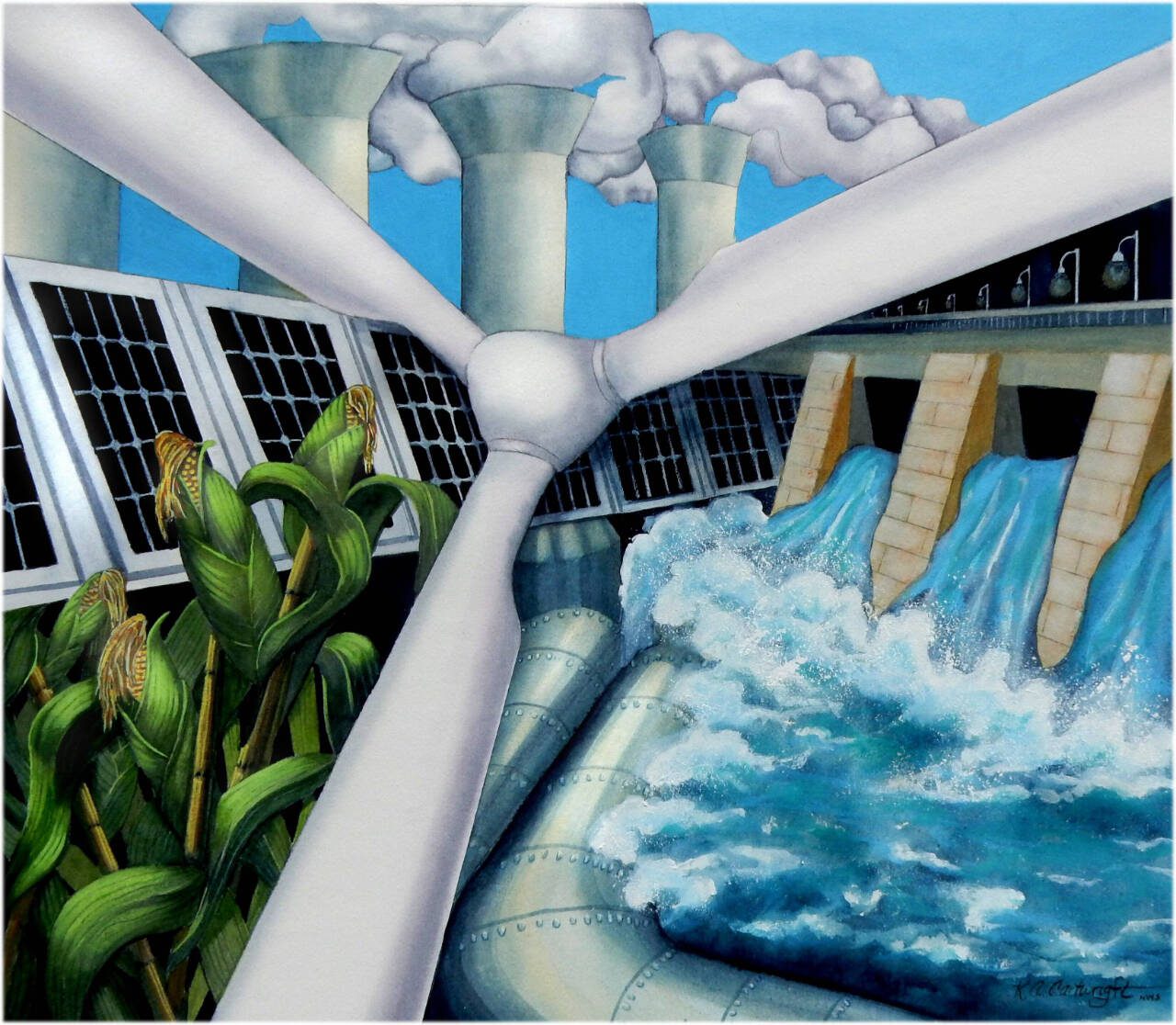The image is a digitally rendered illustration depicting various forms of energy production. At the very center stands a large white wind turbine with its blades extending towards different points of the drawing. One blade reaches towards the top left, another extends to the top right, and a third points downwards towards the bottom left. Above the wind turbine, smokestacks discharge clouds of smoke, set against a blue sky in the background, suggesting industrial energy sources such as nuclear or coal. To the left of the wind turbine, green corn stalks rise, possibly indicating biofuel production like ethanol. Adjacent to the corn, slightly above, are solar panels capturing sunlight for solar energy. On the right-hand side of the image, a hydroelectric dam is depicted with vibrant blue water cascading down its structure, illustrating hydroelectric power. The composition effectively showcases different methods of generating electricity, encompassing wind, solar, hydro, and potentially biofuel and industrial sources, all within a cohesive frame.